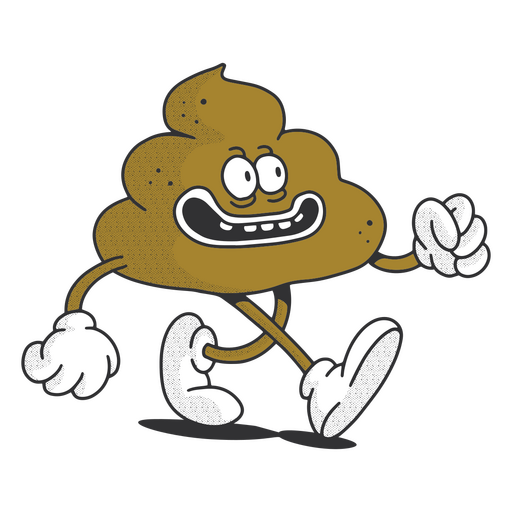The image depicts a cartoonish, anthropomorphic poop emoji, drawn in brown with white accents, placed on a transparent background. The character has a pile-like body with expressive wide, circular eyes and a smiling mouth outlined in white, showing a top row of five spaced-apart white teeth. It features long, skinny arms and legs, each adorned with large, white cartoon gloves that have four fingers, and oversized white shoes. The figure appears to be in mid-motion, as if walking, with one foot slightly off the ground while the other foot's heel is lifted, casting a shadow below. The character is facing to the right, with the right arm extended upwards and the left arm extended downward, suggesting it is engaging in an enthusiastic strut.